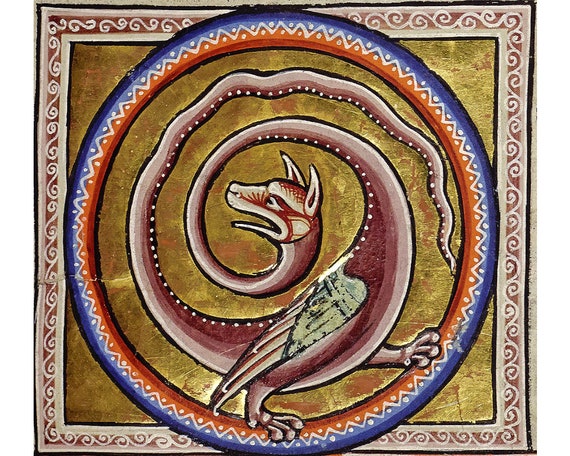This square rug showcases an intricate and colorful design. At its core, a prominent blue and red circle extends to the edges, surrounded by a vibrant background of gold. Encircling this central motif is a decorative rim featuring white, swirling lines that form a series of V-shaped patterns, each adorned with white dots at their peaks and troughs. Beyond this, a secondary border displays alternating red and tan with delicate swirls.

At the center of the circle resides a fantastical creature, blending elements of various animals: it has the face of a wolf with long, pointy ears, a body reminiscent of both a dragon and a bird, and a serpentine tail. Its long, thin neck leads to a partially open mouth, giving it a dynamic appearance as if caught in motion. The creature's body includes a large feathered wing, though it's not particularly expansive, and it stands on two mammalian hind legs, one positioned directly beneath it and the other stepping forward. All of this is enveloped by a dual-color ring, red and blue, that features decorative white lines and dots, enhancing the rug's vivid and historic aesthetics. The creature itself is a mix of purple and black hues, with wings tinged greenish-black, resulting in a striking focal point that captures the eye.